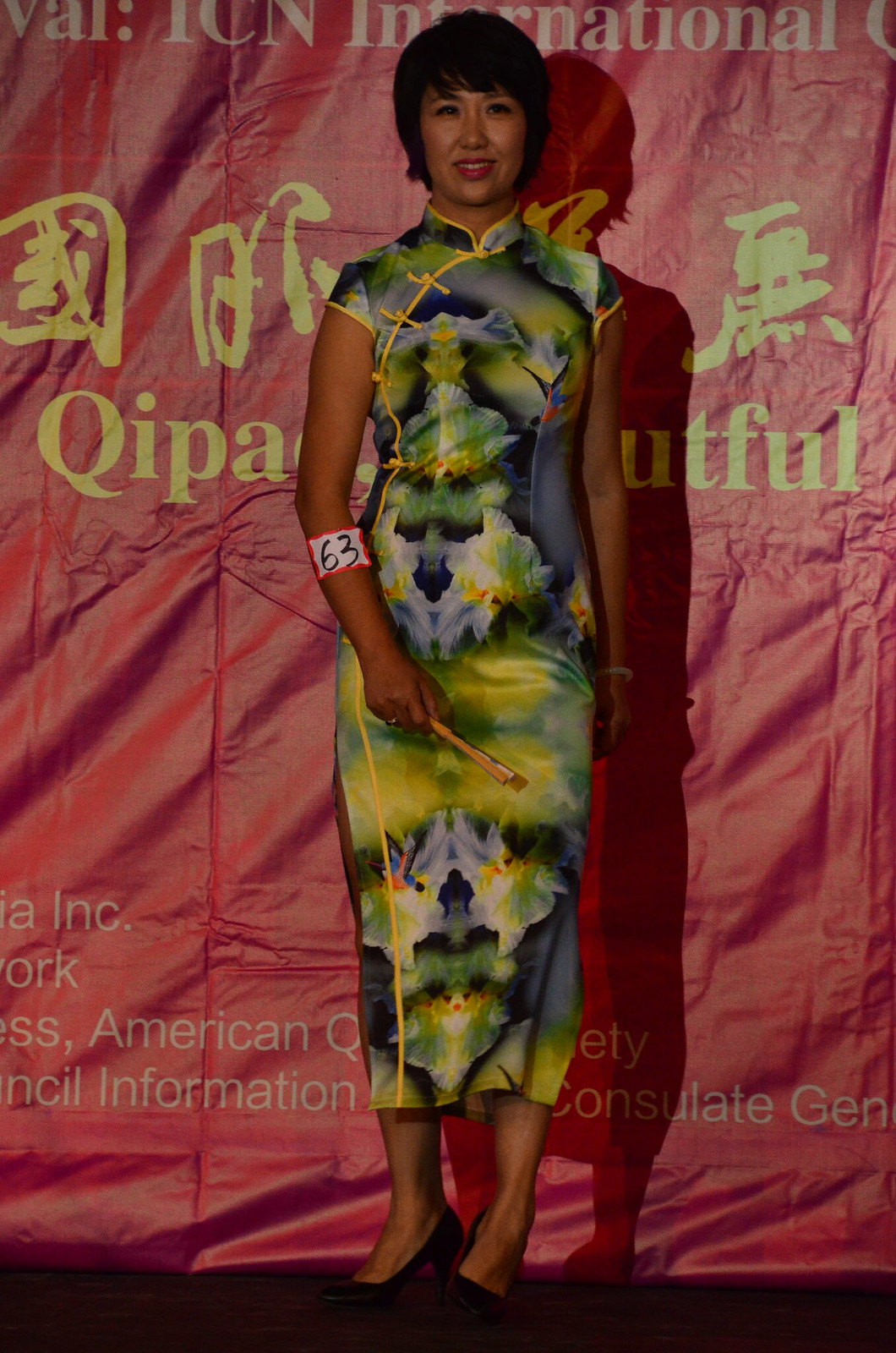In this image, a woman of Asian descent stands at the center, looking directly at the camera. She is dressed in an elaborate kimono-style dress that features a harmonious blend of green, blue, and yellow, adorned with a floral pattern. A distinctive yellow strip runs from her neckline down the side of her body to her leg. On her forearm, she wears a sticker displaying the number 63. She holds a traditional fan, adding a cultural touch to her attire. Behind her, a partially obscured sign reveals the letters "Q-I-P-A," suggesting she might be participating in a beauty contest or cultural event, though the exact context is unclear. The setting is indoors, with the woman positioned centrally against a backdrop that appears to be fabric, contributing a variety of colors including brown, pink, white, light green, yellow, blue, orange, gray, gold, and another yellow. The floor seems to be hard, possibly carpeted, further hinting at a formal or staged environment like an awards show.